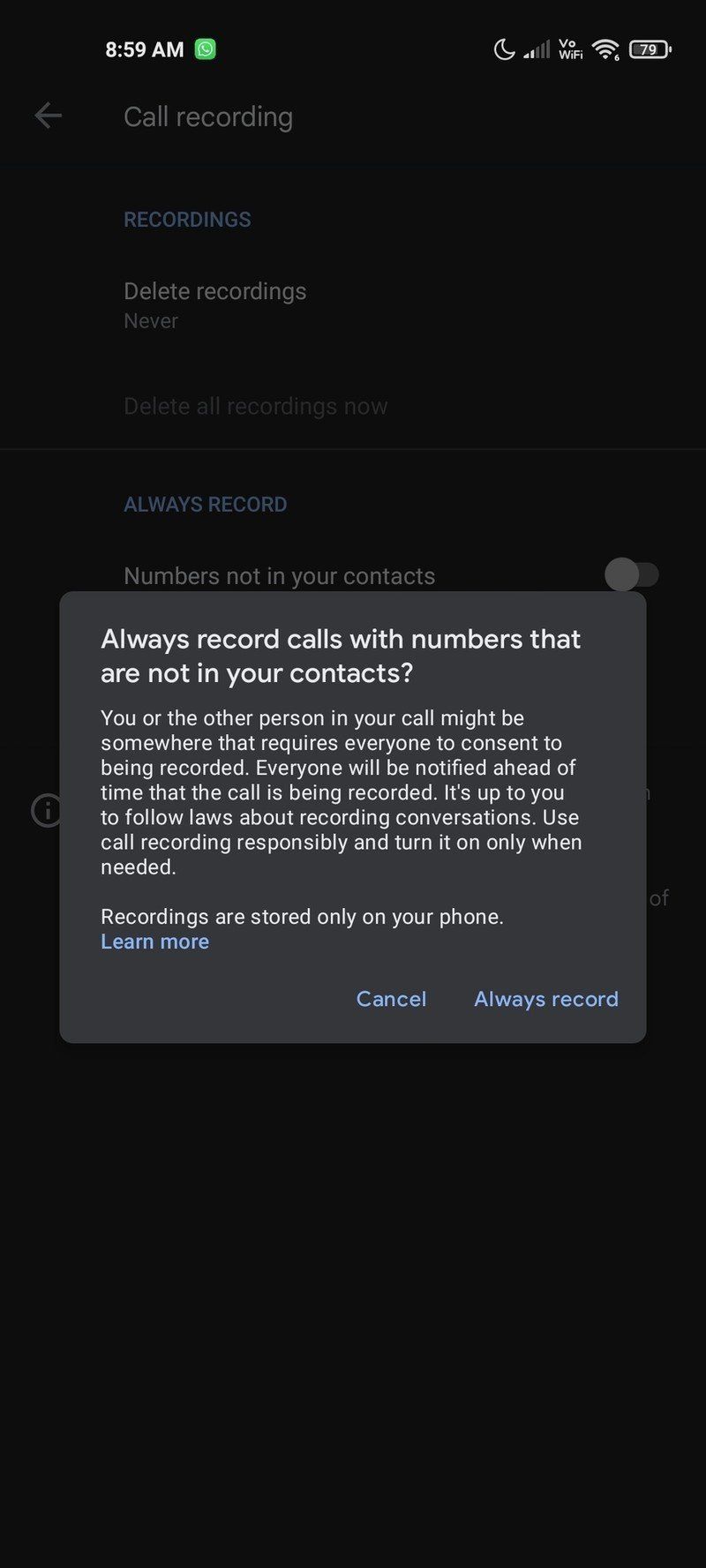This is a detailed screenshot of a phone display regarding call recording settings. The screenshot features a predominantly black background with various elements visible on the screen.

At the very top, the status bar displays the current time as 8:59 a.m. in white numerals. To the left of the time, there's a small green square with a phone icon inside, indicating an active call. Further left on the status bar, you can see indicators for signal strength, Wi-Fi strength, and a battery level at 79%.

Below the status bar, in light gray text, the phrase "Call recording" is prominently displayed with a back arrow pointing to the left, suggesting an option to navigate back. 

Central to the screenshot is a prominent pop-up box with a dark gray background and white text. The text reads:

“Always record calls with numbers that are not in your contacts?
You or the other person you call might be somewhere that requires everyone to consent to be recorded. Everyone would be notified ahead of time that the call is being recorded. It’s up to you to follow laws about recording conversations. Use call recording responsibly and turn it on only when needed. Recordings are stored only on your phone.”
 
Below this text is a “Learn more” link. 

At the bottom of the pop-up box, there are two clickable options in blue text: “Cancel” and “Always record”.

Additionally, the screenshot shows other options related to call recordings against the black background:

- Recordings
- Delete recordings
- Never delete all recordings
- Always record numbers on your contacts (with a toggle switch)